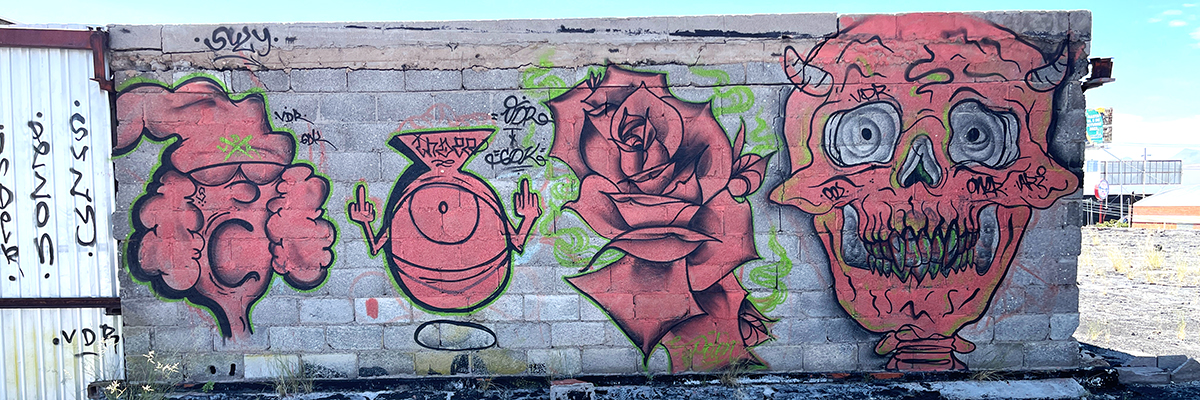This digital image, captured outdoors during the daytime, showcases a grey brick wall adorned with intricate graffiti artwork. The wall features four prominent illustrations in shades of light red and pink, accented by green halos. Starting from the left, the first image is a cartoonish character with curly hair, glasses, an open mouth, and a Santa-like hat, caught in mid-yell. Next to it is a quirky round character with a single large eye, defiantly flipping off the viewer with both hands. The third illustration is a meticulously detailed rose with vibrant petals. Finally, to the right, there is a stylized skull head adorned with small horns protruding from its forehead. The scene is framed by a bright blue sky, a large building featuring extensive glass windows, barren earth, and sparse patches of light green grass.